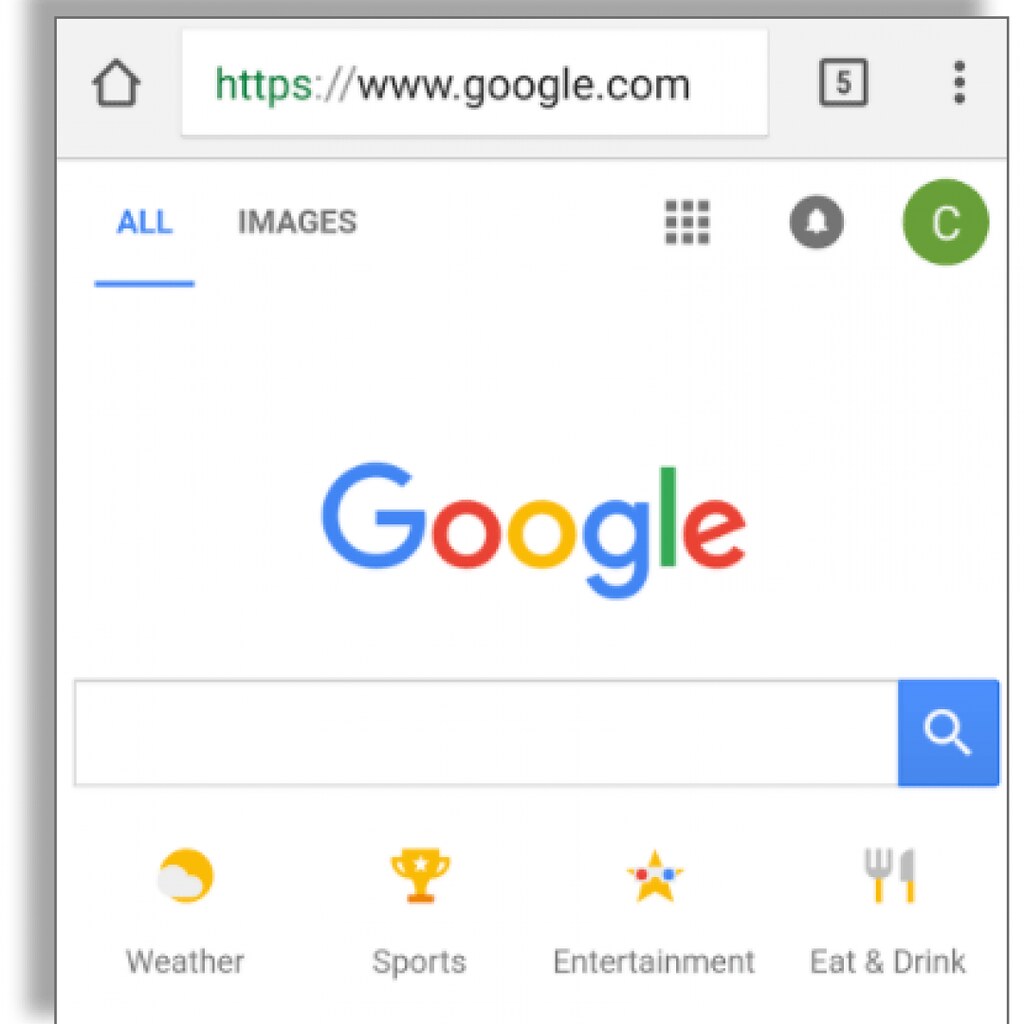The image appears to be a screenshot of the Google homepage displayed on a mobile device. The top section features a gray navigation bar, which includes a house icon on the left, symbolizing the home screen. To the right of the home icon is the URL field, displaying "https://" in light gray, followed by "www.google.com" in darker gray. Adjacent to the URL on the right, there is a number "5" enclosed in a square, along with three vertically aligned dots that likely represent additional options. This entire segment is set against a light gray background.

Moving down, a horizontal line separates the gray bar from the white background below. On this white background, the word "All" is highlighted in blue and underlined, indicating the current selection, next to "Images." To the right, there is an icon made up of nine small squares forming a larger square, a bell icon within a circle, and a green circle enclosing a white letter "C."

Centered on the page is the multicolored Google logo, with each letter in a different color (blue, red, yellow, blue, green, and red). Beneath the logo is an empty Google search bar, which features a blue button with a white magnifying glass icon on its right end. The search bar itself is outlined in gray.

Below the search bar are various category options in gray text: "Weather," "Sports," "Entertainment," and "Eat and Drink." Each category is accompanied by an icon: a cloud with a sun for Weather, a trophy for Sports, a star for Entertainment, and a knife and fork for Eat and Drink.